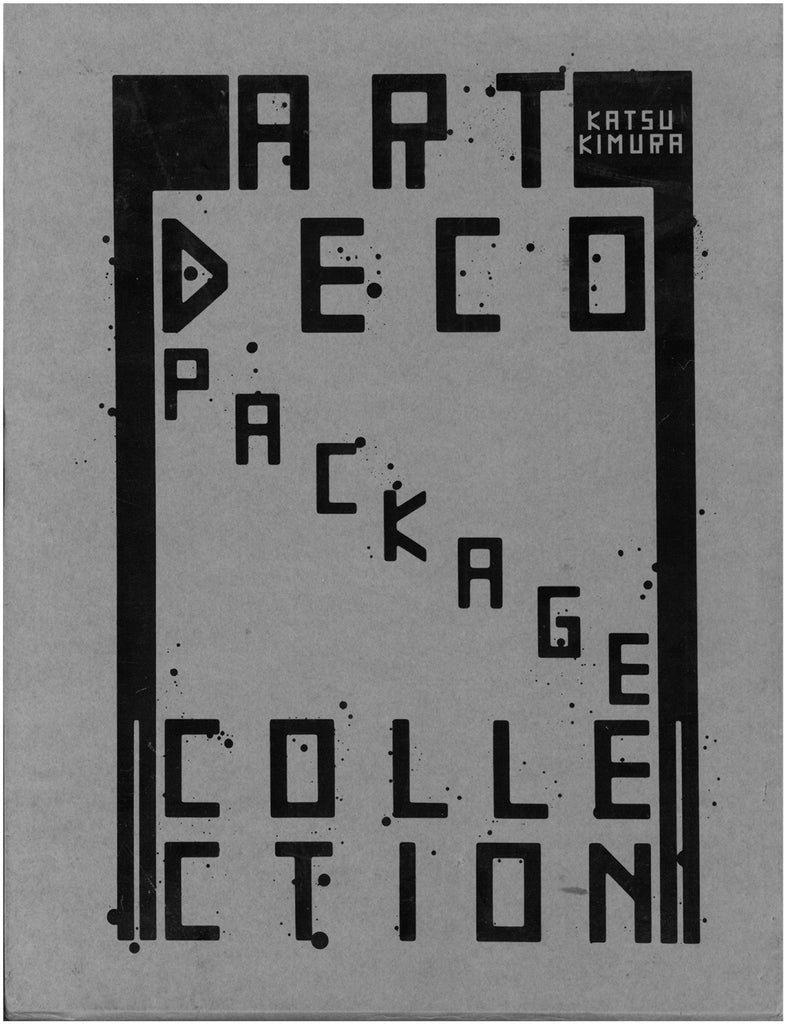This striking black-and-white image employs a highly stylized Art Deco font, featuring bold geometric designs and intricate trimming. At the top of the image, the word “ART” stands prominently, followed by “DECO” beneath it. Positioned diagonally across the image, the word “PACKAGE” creates a stair-step pattern leading from the upper left to the lower right. The terms “CALAIS” and “SEYCHELLES” are displayed underneath. The border is accentuated with bold black lines and geometric patterns characteristic of the Art Deco style. In the upper right corner, within a black square that blends seamlessly into the border, the name “KATSU KIMURA” is inscribed in the same distinctive font, indicating perhaps the artist or designer behind the work. Scattered throughout the image are small splatters of black ink, adding an element of the unexpected to the otherwise structured design. Overall, the image exudes a meticulously crafted Art Deco aesthetic, likely representing an "Art Deco Package Collection."